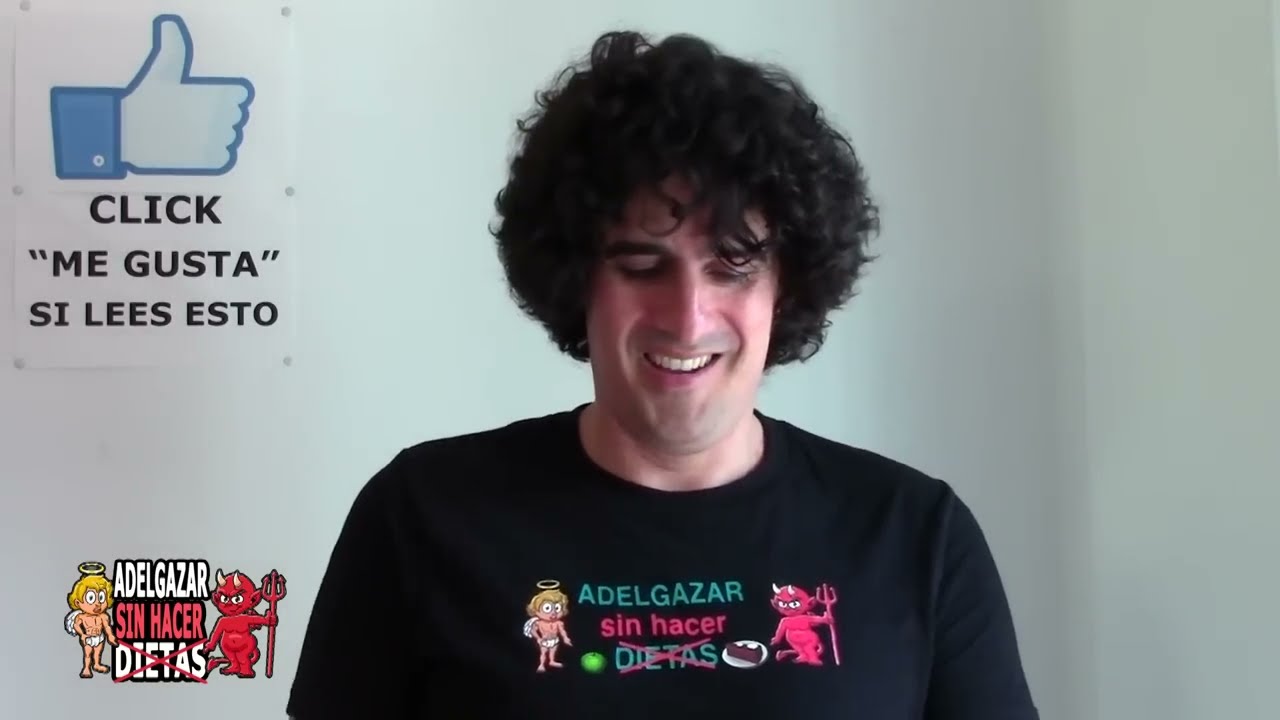In the image, we see a Caucasian man, likely in his late 20s or early 30s, with dark brown, bushy, curly hair that falls to the nape of his neck. He is slightly smiling with upturned corners of his lips, revealing the top row of his teeth. His elongated face and straight nose are noticeable. He is looking downward, possibly at something in his hands. 

He is wearing a black T-shirt adorned with several Spanish words and illustrations. Prominently in blue letters across the front of the shirt is "ADELGAZAR". Below that, in red letters, is "SIN HACER", followed by "DIETAS" in blue-green letters with a red cross through it. On the left side of these words is a small angel illustration, wearing white underwear, with blonde hair, a gold halo, and white wings. On the right side is a red devil figure holding a pitchfork. This same angel and devil duo reappear on the lower left side of the shirt with the same words between them: "ADELGAZAR" in white, "SIN HACER" in red, and "DIETAS" in white with a red cross through it.

In the background, which is entirely white, there is more text and imagery. In the upper left corner, there is a blue thumbs-up emoji. Below that, in black letters, it says "Clic Me Gusta Si Lees Esto," which translates to "Click Like if You Read This." Additionally, a gray background appears alongside the repeated illustrations and text, reinforcing the angel and devil motif and the same Spanish phrases: "ADELGAZAR, SIN HACER, DIETAS." On a table next to the man, there is also a green apple.

Overall, the image portrays a consistent theme of visual and textual elements repeated across different sections, emphasizing the interplay between the angel and devil figures with the phrases related to weight loss and dieting in Spanish.